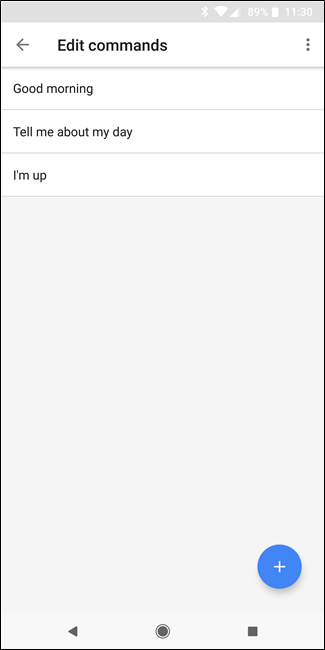The image displays a smartphone interface with a gray rectangular notification bar at the top, outlined in black. On the top right-hand side of this bar, a series of symbols are arranged from left to right: a Bluetooth symbol, a Wi-Fi signal icon with increasing lines, a "99%" battery life indicator, and finally a battery icon. Below this bar is a white rectangle showing the time "11:30".

Beneath the time display is a white rectangle with an arrow pointing left, labeled "Edit Commands." Next to this label, on the far right-hand side, are three vertical dots indicating additional options.

Below this command section are three areas separated by thin gray lines:
1. The first section is labeled "Good Morning."
2. The second section is labeled "Tell me about my day."
3. The third section is labeled "I’m up."

The rest of the screen appears mostly blank until the bottom. At the lower right corner, there is a prominent blue circle with a white plus sign inside, partially overlapping a gray rectangle pointing left. Next to this rectangle is a circular gray icon outlined with an inner gray circle, followed by a small gray square.

In summary, the interface showcased consists of various sections for notifications and commands, organized neatly with clear labels and icons.